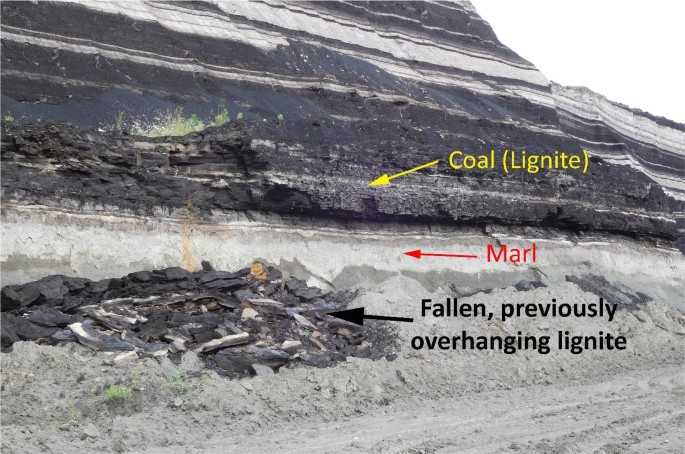The image appears to be a detailed, cross-sectional illustration of a rock formation or hillside, serving an informational purpose. The top section features shiny black stone with white stripes, highlighted by a yellow arrow pointing down to the bottom left, marked with the yellow text "COAL (LIGNITE)." Below this, a red arrow points horizontally to the left, indicating a middle layer of gray stone labeled "MARL" in red letters. At the base of the formation, near the left, a thick black arrow points towards an area of fallen rubble, annotated with the black text "FALLEN, PREVIOUSLY OVERHANGING, LIGNITE." The colors in the image include various shades of gray, white, yellow, red, black, and a hint of green, with a white sky in the upper right corner. This illustration provides a detailed depiction of the layered sediment and rock formation, emphasizing the coal and lignite's structural behavior within the hillside.